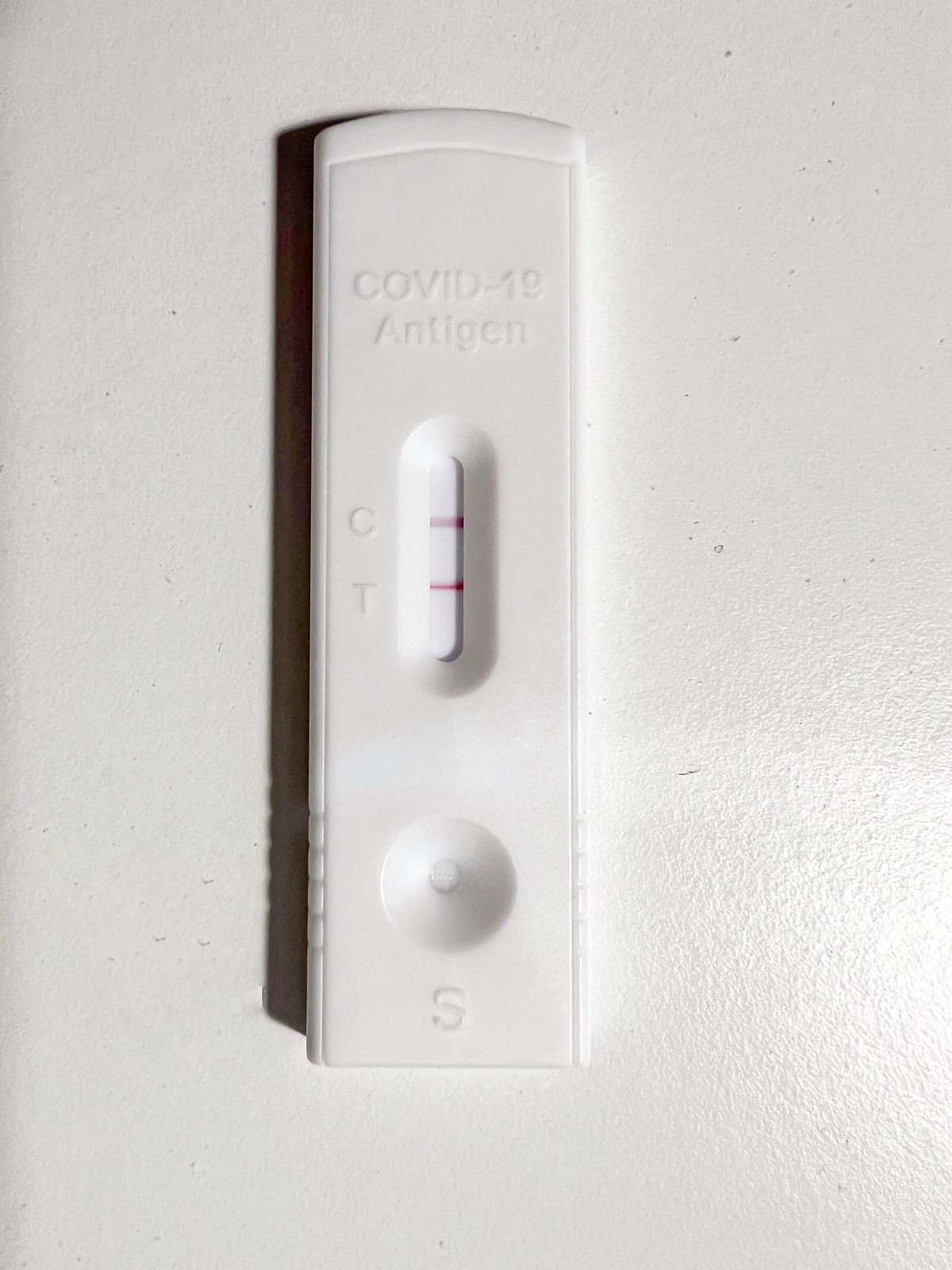In the photograph, a COVID-19 test strip is prominently displayed against a white, slightly textured tabletop. The test strip, which is also white, bears the words "COVID-19 Antigen" near the top. Just beneath this text, there is a small window with two visible red lines, signifying a positive test result. The upper line, marked with a "C" indicating the control line, and the lower line, marked with a "T" indicating the test line, both confirm the presence of the virus. Below the window, you can see a circular opening labeled with the letter "S." The whole test strip casts a subtle shadow to its left, adding a touch of dimension to the composition.